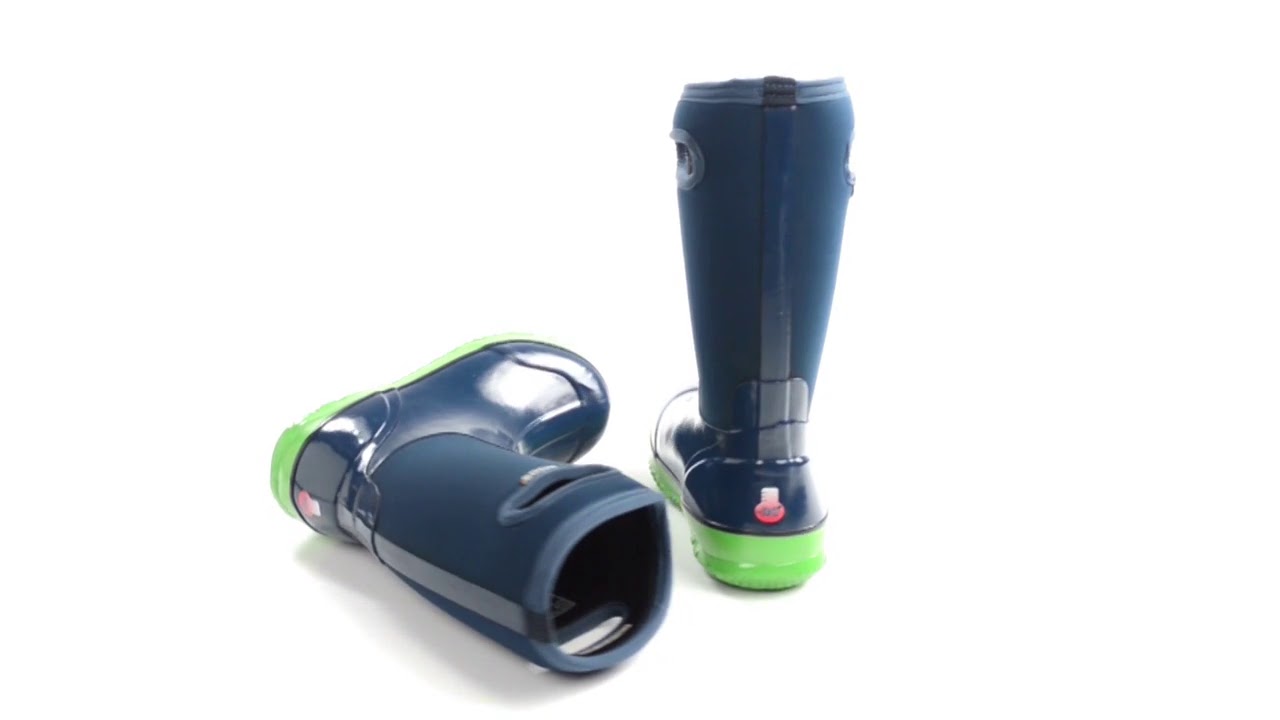This image features a pair of high rubber boots designed for wet or muddy environments. The boots are primarily dark blue with different materials for the upper and lower sections, suggesting sturdiness and durability. Each boot has neon green soles that provide a striking contrast and appear to wrap around the bottom rim. Notably, the boots are adorned with lighter blue accents: there is a strip running vertically down the back and reinforcement on the toe and heel. The right boot stands upright, facing slightly away from the viewer, while the left boot is lying on its right side, toes pointing outward at an angle. Both boots feature convenient hand openings at the top for easy pull-on. Additionally, there is a unique emblem or sticker on the back heel, predominantly white and red, shaped with a circular bottom and a square top. The boots' interiors appear to be black, enhancing their waterproof design.